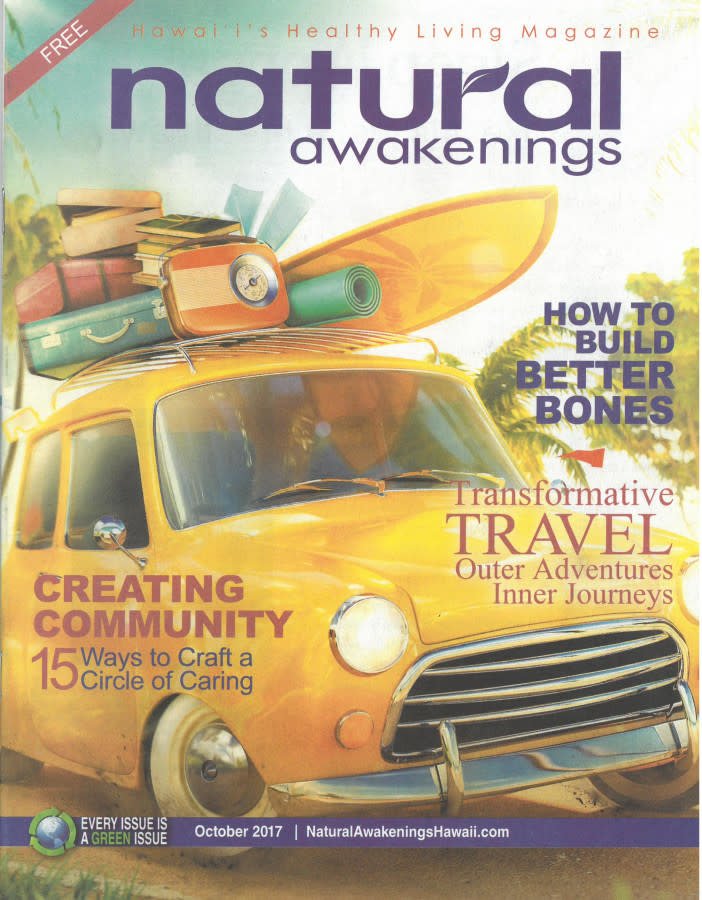The cover of the October 2017 edition of *Natural Awakenings* magazine, labeled as a "Wise Healthy Living Magazine," features a tropical-themed illustration of a small yellow car on a dark road framed by grass. The car, depicted on an island setting with palm trees and a sunny sky in the backdrop, is laden with travel gear atop a metal rack: a partially open suitcase with a clock inside, a bedroll mat, several books tied together, a surfboard, and flippers. The car's interior, visible and blue, appears empty.

In the top left corner, a diagonal label proclaims the magazine as "Free." Dominating the upper portion, in large blue lettering, is the title "Natural Awakenings," featuring a leaf motif. To the right of the car, text in blue reads "How to Build Better Bones." Beneath it, in red, is "Transformative Travel," followed by "Outdoor Adventures, Inner Journeys" in subsequent lines. On the left-hand side, aligned vertically, it reads "Creating Community" in large red letters, with "15 Ways to Craft a Circle of Caring" in smaller black text. A banner spans the bottom: "Every Issue is a Green Issue," along with "October 2017" and the URL "naturalawakeningshawaii.com." The cover also includes a globe graphic encircled by green arrows, reinforcing the magazine's eco-friendly theme.